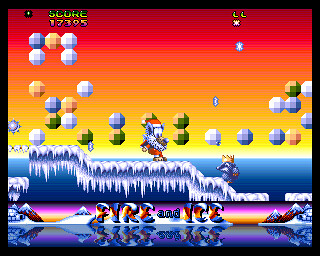The image is a vibrant screenshot from the classic computer game "Fire and Ice," which appears to be from the 1980s. The bottom 10% of the image features a colorful banner displaying the game's title: "FIRE AND ICE." The words "FIRE" and "ICE" are in bold uppercase, with "FIRE" in red and "ICE" in blue, while the word "and" is in lowercase blue lettering. The banner also includes an igloo and mountain scene at both ends, producing a mirror-like reflection beneath it, as though it's perched above water.

Above this banner, the main game screen unfolds. It showcases a snowy, icicle-covered walkway that descends from left to right. At the center of the screen stands the protagonist, resembling Sonic the Hedgehog but distinguishable by his red hat and a red coat adorned with a sheepskin collar. Below him on the walkway, a mole-like creature with a golden crown gazes upwards. Scattered throughout the air are various octagonal, multi-colored blobs, likely collectible items within the game.

At the top left corner of the screen, the player's score reads 17,395. The background portrays a stunning sunset gradient, transitioning from red to orange and yellow hues as it descends.

This rich tapestry of details not only visually delights but also captures the essence of retro gaming nostalgia.